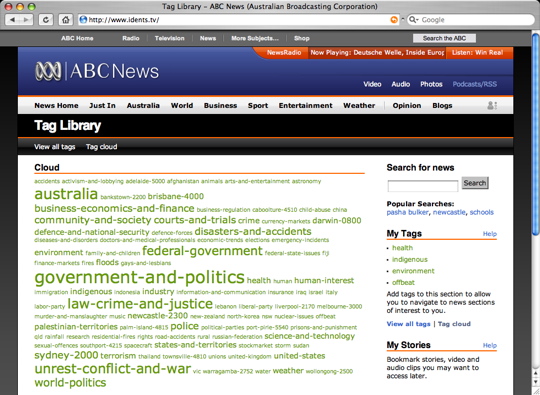This screenshot captures an older web browser interface, likely Internet Explorer from the mid to late-2000s, evidenced by its gray color and vintage web design style. At the very top, the browser window displays the title "Tag Library ABC News (Australian Broadcasting Corporation)," indicating that this is the ABC News website from Australia.

Directly beneath the browser's title bar, there's a horizontal gray menu bar featuring links to "ABC Home," "Radio," "Television," "News," "More Subjects," and "Shop." Below this, the main header is a solid blue color. On the left side of this header, "ABC News" is written in a very light gray font, accompanied by a logo resembling interconnecting rings or a spiral.

Another menu is placed beneath the blue header, with a light gray background and black font. This menu includes categories such as "News Home," "Just In," "Australia," "World," "Business," "Sport," "Entertainment," "Weather," "Opinion," and "Blogs."

Following this, in a black background section, the term "Tag Library" is prominently displayed. The final section of the screenshot is a white background area showcasing various tags in a word cloud format. The most frequently used tags, appearing larger, include "Australia," "Government and Politics," "Federal Government," "Law," "Crime," and "Justice," "Sydney 2000," "Unrest, Conflict, and War," and "World Politics."